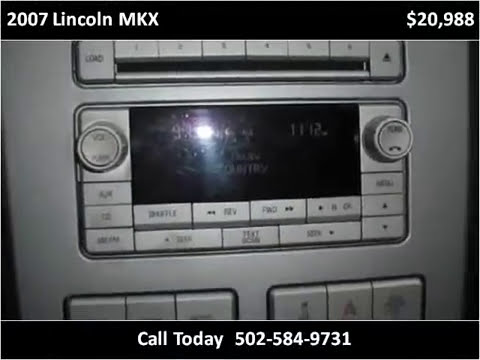The image features the detailed view of a car stereo system embedded within the dashboard of a 2007 Lincoln MKX. The stereo is housed in a silver panel adorned with an array of silver buttons, including functions like shuffle, rewind, forward, alarm, phone, volume, load for CD player, play, and eject. The central section showcases a dark screen with a small reflection of light. On the top bar of the image, white text reads "2007 Lincoln MKX" with a price tag on the upper right corner stating "$20,988." At the very bottom, there is another black bar with white text prompting viewers to "Call Today" followed by the phone number 502-584-9731, indicating it might be from an old advertisement.